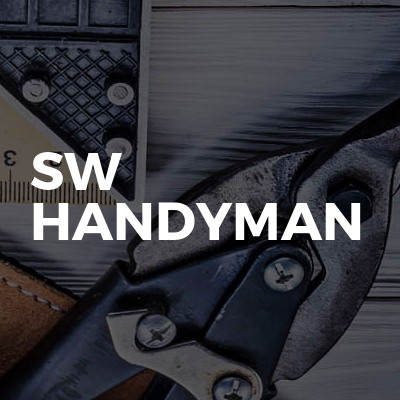The image is a designed square box, reminiscent of a card format seen on websites or blogs, showcasing a visual representation centered around handyman tools. The central focal point is white block text, all capitalized, with "SW" on the first line and "HANDYMAN" beneath it. The text is left justified and stands out prominently in the middle of the image, overlaid on a semi-transparent black filter that dims the photograph behind it. The photograph features a collection of various tools arranged on what appears to be a gray wooden tabletop, with noticeable wood grain. To the upper left, there is a ruler and possibly a set square, highlighting precise measurements. The bottom right showcases metal garden hedge trimmers with a triangular hinge held by three screws, leading into sleek silver blades. A piece of brown leather with gray stitching is visible in the lower left, and a tool resembling bolt cutters with a blue handle is also present. The background's cohesive display of tools hints at craftsmanship and precision, adding depth and texture to the visual narrative.